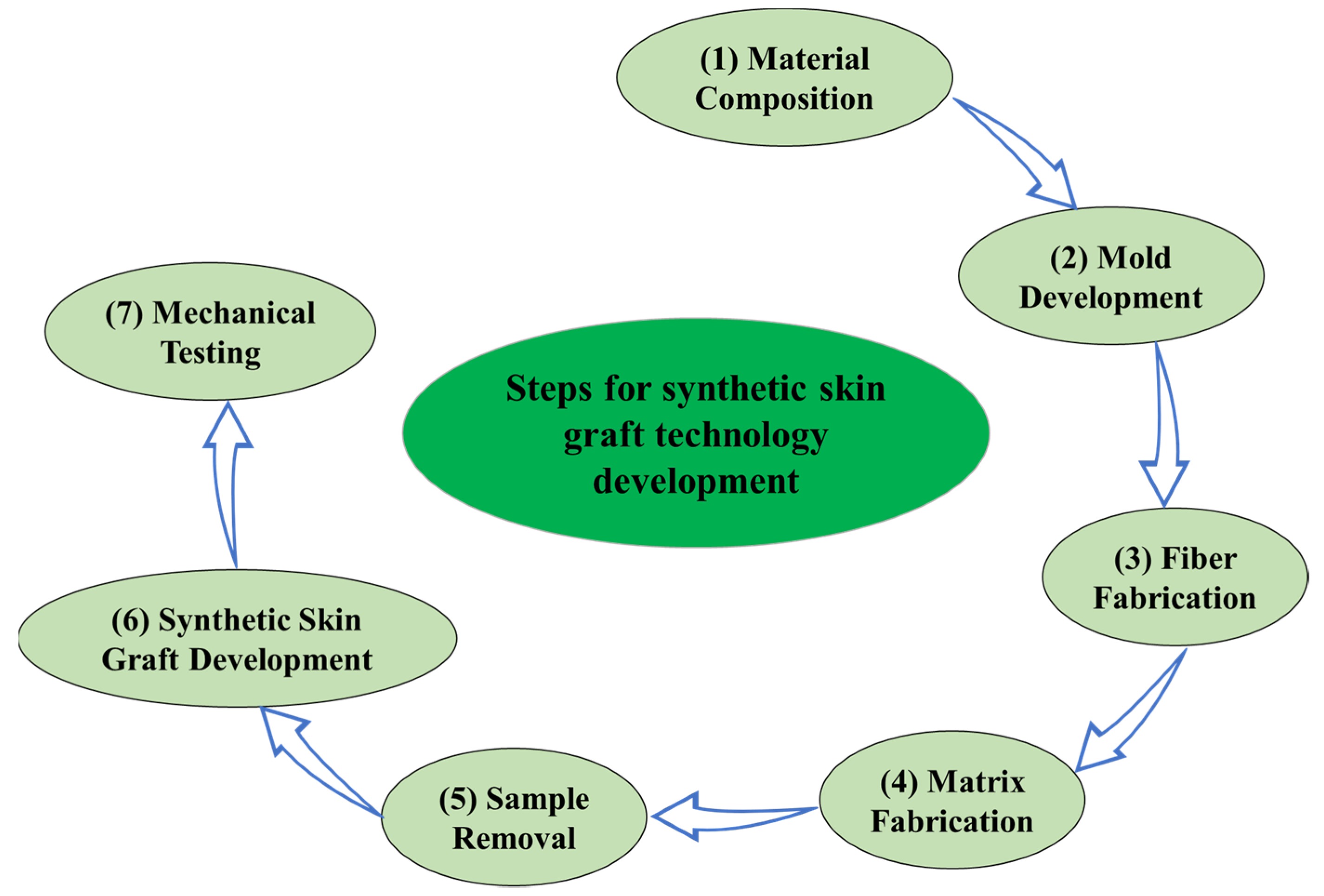This detailed digital drawing illustrates the steps involved in synthetic skin graft technology development. At the center of the image, a green oblong shape contains the title "Steps for Synthetic Skin Graft Technology Development" in black lettering. Surrounding this central shape are light green ovals each containing a step, starting at the upper right with 1. Material Composition, then proceeding clockwise with blue arrows to 2. Mold Development, 3. Fiber Fabrication, 4. Matrix Fabrication (positioned around the bottom), 5. Sample Removal, 6. Synthetic Skin Graft Development, and finally 7. Mechanical Testing. The diagram utilizes a color scheme of green, light green, black, and blue to clearly indicate the progression of each step in the synthetic skin grafting process.